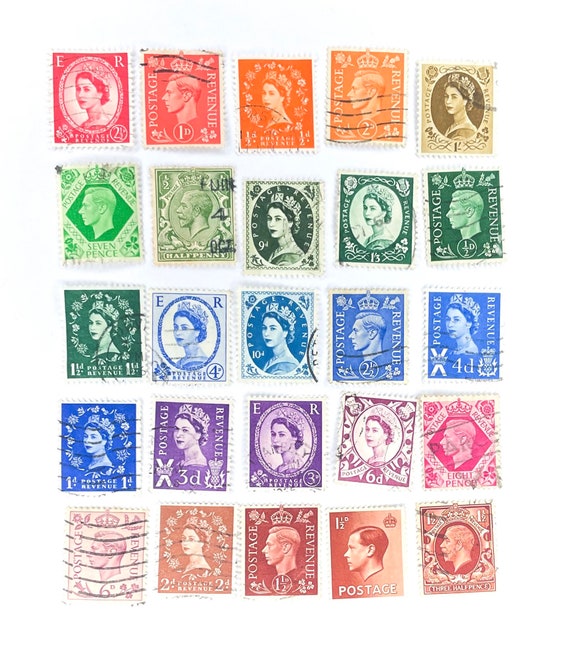This color photograph showcases a meticulously organized array of 25 British postage stamps, arranged in a 5x5 grid against a white background. Each row of stamps is color-coordinated, starting with pink and orange in the top row, followed by various shades of green in the second row, transitioning to blue in the third row, purple in the fourth, and finally brown and sepia tones in the bottom row. The stamps predominantly feature images of Queen Elizabeth, with occasional depictions of previous monarchs. They display various denominations, including 1D, ½D, 4D, and 3D, and many bear postmarks, reflecting their historical use. This carefully curated collection captures the diversity and history of British postage.